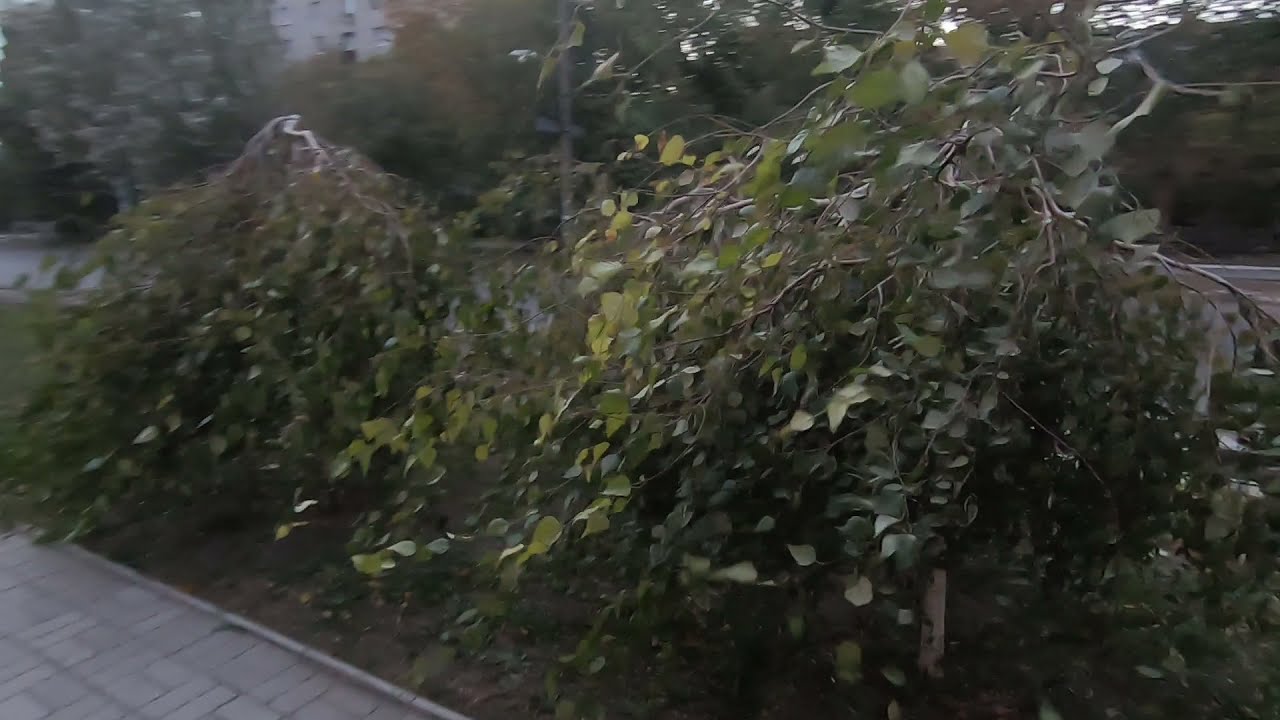In the foreground of the image, two scraggly, large bushes, approximately two and a half to three feet tall and about a foot wide, dominate the scene with their abundant thin green leaves. Between and partially obscuring the bushes, a glimpse of dirt or mulch is visible on the ground, along with a small portion of brick-like sidewalk or curb area. The foliage appears overgrown and untamed, with branches hanging loosely, resembling the unkempt aspect of weeping willows. Beyond these bushes, the background reveals an obscured roadway, flanked by blurry trees and additional bushes. The image, taken outdoors, has a blend of greens, browns, and grays, with lighting that suggests it might be around sunrise or sunset. Further back, past the main bushes, more vegetation is discernible, including small ornamental trees, though they remain out of focus and indistinct.